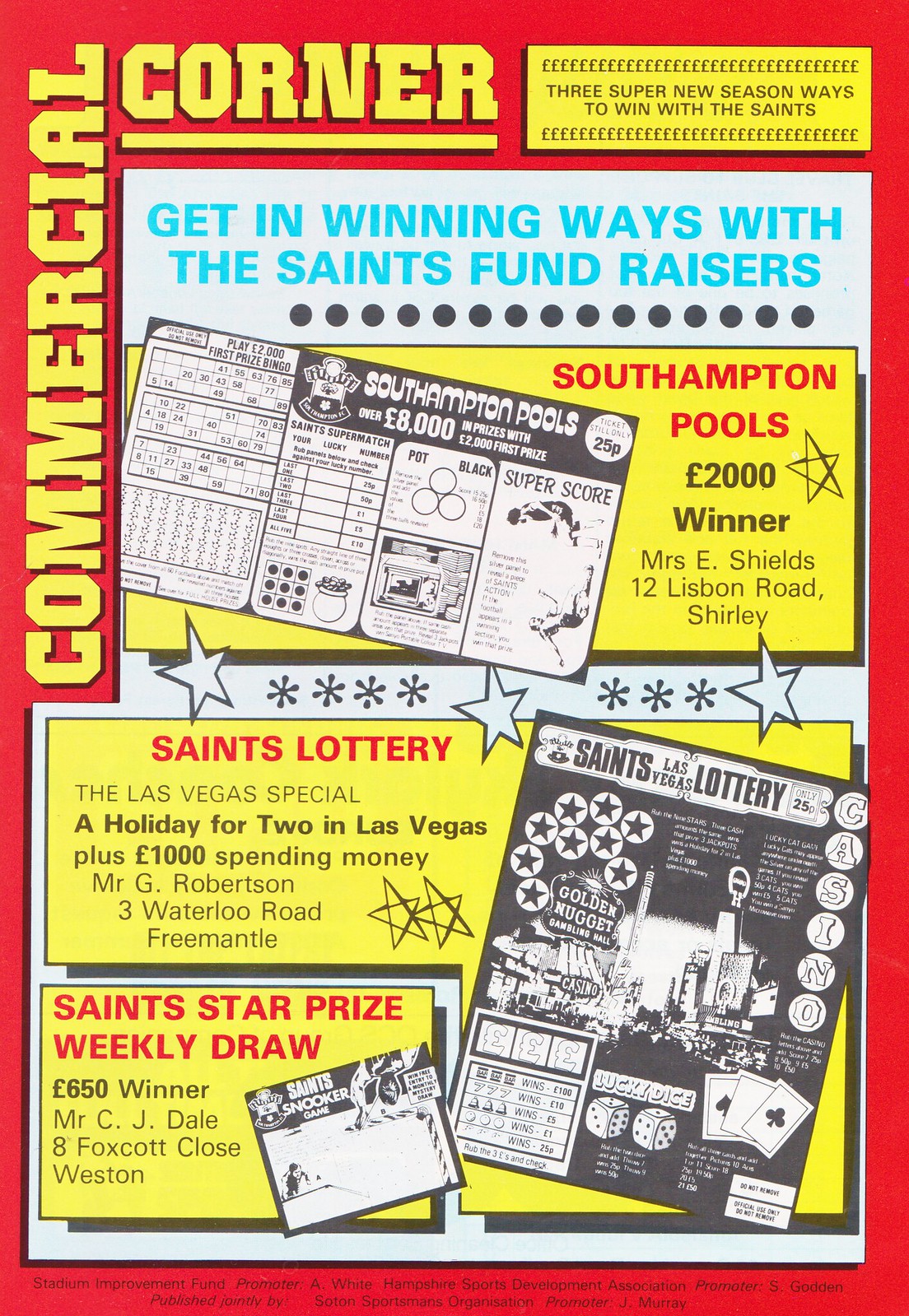This image is the front cover of a magazine feature titled "Commercial Corner," which focuses on advertisements. It has a vibrant design with a red background and various white and yellow boxes containing text. The primary color scheme consists of black text on yellow backgrounds, framed by a red border, giving it an eye-catching appearance.

Prominently displayed are images of scratch tickets and puzzle tickets, indicating themes of games and prizes. At the top right corner, in a yellow box with black text, two lines read: "3 Super New Season Ways to Win with the Saints." 

The featured promotions include:
1. **Southampton Pools**:
   - Prize: £2,000
   - Winner: Mrs. E. Shields, 12 Lisbon Road, Shirley
   - Highlight: A star symbol is drawn next to this information.

2. **Saints Lottery - The Las Vegas Special**:
   - Prize: A holiday for two in Las Vegas plus £1,000 spending money
   - Winner: Mr. G. Robertson, 3 Waterloo Road, Freemantle
   - Highlight: Two stars are drawn next to this information.

3. **Saints Star Prize Weekly Draw**:
   - Prize: £650
   - Winner: Mr. C. J. Dale, H. Foxcott Close, Weston